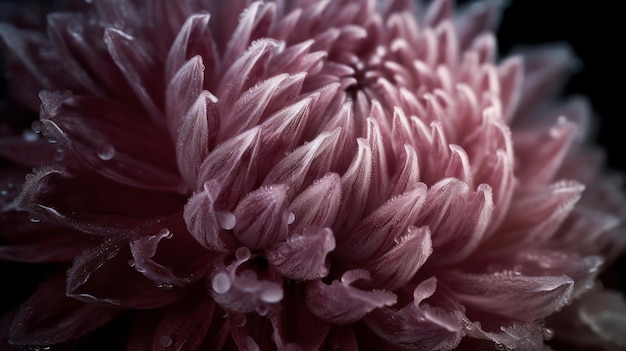This image showcases an extreme close-up of a fully bloomed pink chrysanthemum, capturing intricate details that blur the lines between a photograph, digital painting, or AI-generated art. The chrysanthemum, centered against an indistinct, dark background, displays an abundance of petals, each with pointed oval shapes. The petals are coated with dew droplets and, notably, some exhibit ice-like formations, particularly on the left side of the flower. This suggests the chrysanthemum experienced a chilly night. The outer petals splay outwards as you move away from the densely packed center, which features white-tipped petals adding to its visual allure. The intense focus of the image reveals the flower's layered structure and the reflections from the water droplets, making the petals appear almost fuzzy, soft, and vividly detailed.